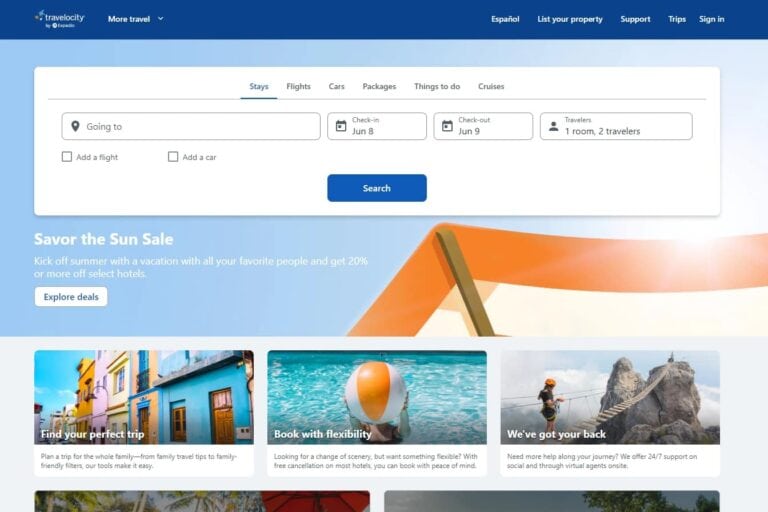The Travelocity website features a distinctive blue navigation bar at the top, displaying options including "More travel" with a drop-down menu, a language toggle button labeled "Español" to switch the site to Spanish, "List Your Property," "Support," "Trips," and "Sign In." The main page is highlighted by an inviting visual of a clear blue sky paired with a cabana or umbrella, evoking a tropical vacation vibe. The promotional text encourages visitors to "Savor the Sun Sale," suggesting they "kick off summer with a vacation with all your favorite people" and mentions offers of "20% off or more on select hotels," along with a prominent white "Explore Details" button.

Below the main banner, the site offers an all-in-one booking section where users can arrange hotels, flights, and car rentals. The current focus is on hotel stays, where users are prompted to input their destination, check-in and check-out dates, and the number of guests. Scrolling down further reveals additional sections like "Find Your Perfect Trip" and "Book with Flexibility," accompanied by various photographs ranging from serene nature scenes and vibrant cityscapes to a playful poolside moment featuring a woman holding a large beach ball. The overall design is both engaging and user-friendly, aiming to facilitate effortless travel planning for users.